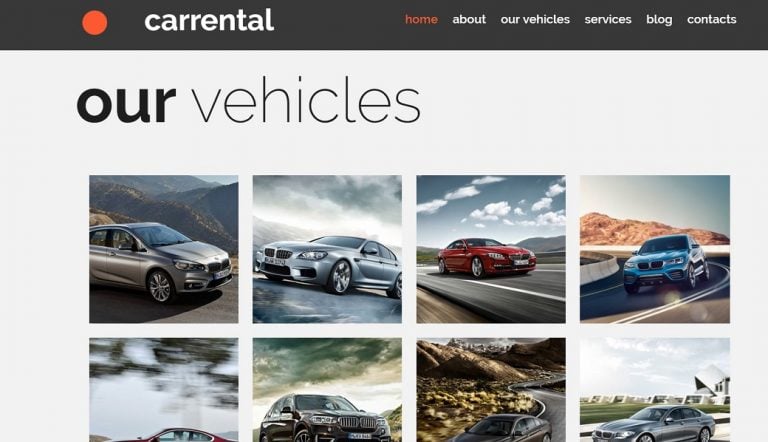This image is a cropped desktop screenshot of a car rental website. The browser and web address are not visible. At the top of the website, there's a black bar with an orange circle, featuring the word "carrental" in white, written as a single word. To the right of this, there are several menu options in orange, displayed in all lowercase letters: home, about, our vehicles, services, blog, and contacts.

The page showcases a section titled "our vehicles," with "our" bolded and "vehicles" not. There are eight vehicle images, though the bottom four are partially cut off. The top four images display:

1. A silver four-door car on a mountainous road.
2. Another silver car driving in a cloudy and mountainous backdrop.
3. A red four-door car on a mountain road under a cloudy sky.
4. A blue four-door car, also set against a mountain background.

The bottom images are less clear:
1. A blurry snippet of what seems to be a red car.
2. A grayish-black car with a cloudy sky.
3. A black car on a road with blurry mountains.
4. A silver car parked in front of what looks like a solar farm.

Overall, the website appears unpolished, suggesting it may be an unfinished sample or draft.